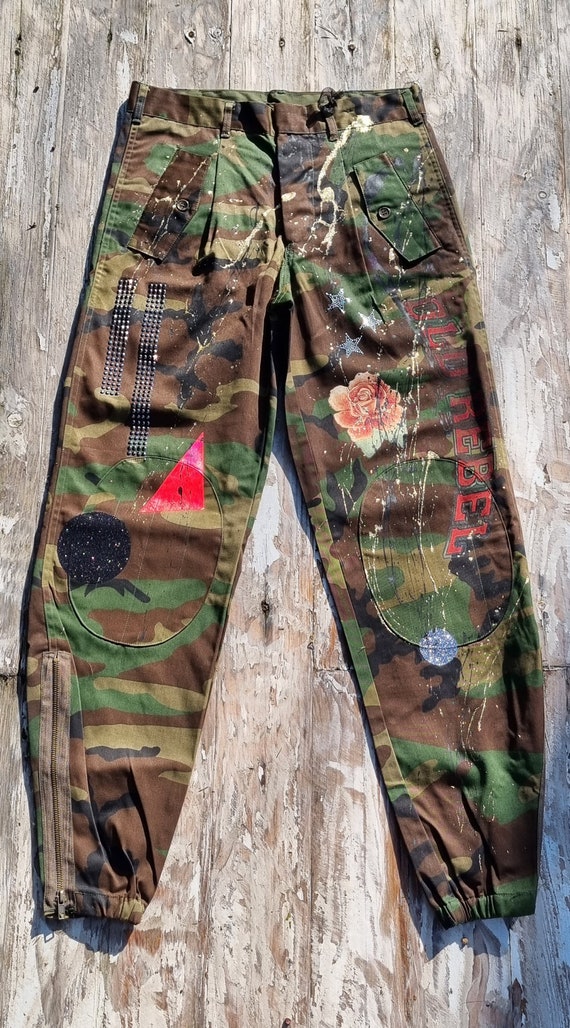The photograph captures a pair of military-style camouflage cargo pants, laid flat on an aged wooden floor characterized by grayish, weathered slats with visible nail holes. The pants are in portrait orientation and show a classic camouflage pattern composed of green, brown, and black hues. The waistline features belt loops suited for threading a belt, while the ankles are gathered with elastic bands and feature side zippers extending up about a foot along the legs. 

The pants are adorned with several distinct patches and artistic elements. Notably, there is a pink rose decal on the top right and a red triangle patch on the left leg, with a black circle positioned below the triangle. Both knees display oblong patches, enhancing reinforcement, with additional white paint splatters scattered across various areas, contributing to a rugged aesthetic. Cargo pockets with flaps are visible near the waist, providing practical storage solutions.

Set against the backdrop of a light grayish wooden surface, possibly a porch or deck, the image was taken outdoors during daylight, presenting a clear, detailed view that emphasizes the product's textured fabric and intricate decor. The style of the image can be described as photographic representationalism, aligned with realism in product photography.